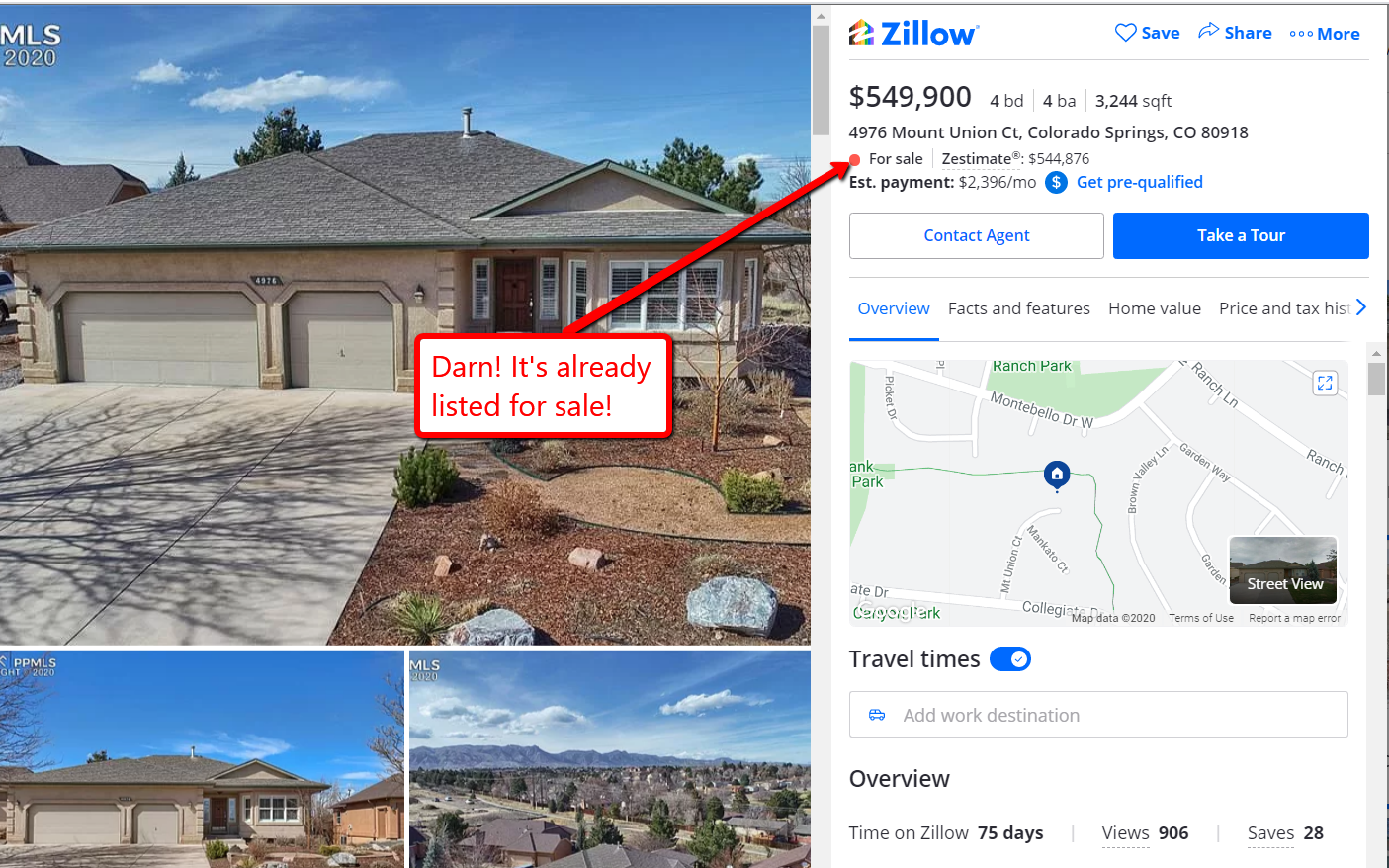Screen capture of a Zillow webpage showcasing a house located in Colorado Springs, Colorado, listed for $549,900. The house features a three-car garage and a xeriscape yard adorned with large rocks and various plants. At the top of the screen, the text "MLS 2020" indicates the image's ownership. Below the main image, additional photos provide different perspectives, including a side view and an elevated shot from a hill that highlights the surrounding neighborhood. The house is described as having four bedrooms and four bathrooms. A caption on the image exclaims, "Darn! It's already listed for sale," reflecting a sense of surprise regarding its availability.